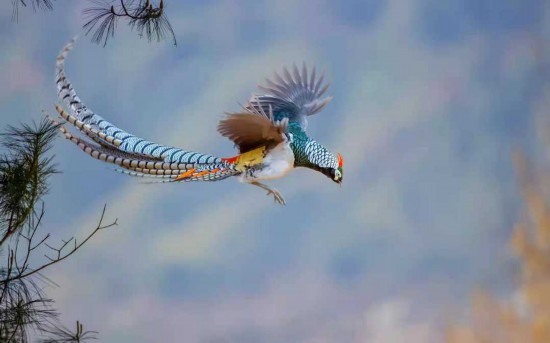In this vivid image captured during the daytime, a unique and ornate bird is shown in mid-flight against a blue sky dotted with white clouds. The bird appears to have just flown off a tree, which is partially visible with branches and needles along the left edge of the picture. On the bottom right, another tree with yellow leaves is visible, though it is blurred and distant. 

The bird is distinctly marked and resembles a small peacock. Its body features a mix of colors including white, yellow, red, and blue. Detailed observations highlight its long blue undertail coverts and black or white and blue markings down its back. The head sports a striking red crest, with a white patch surrounding its eye and a black area under the neck. The beak is a blend of teal, orange, and yellow.

The wings, seemingly gray, are outstretched mid-flight, and the bird's black-and-white striped tail feathers fan out behind it. The intricate detailing of the bird showcases its colorful plumage and dynamic pose, all while it soars towards the right, creating a picturesque and engaging scene.